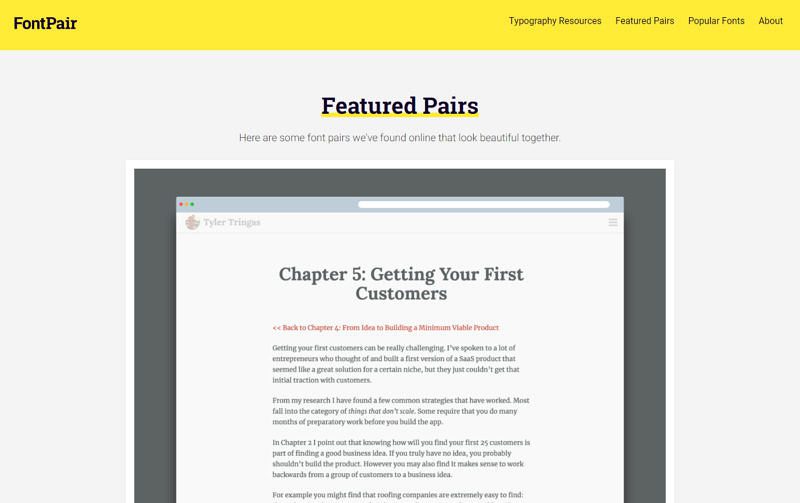The image is a detailed screenshot from a website. At the top, a yellow bar stretches across the screen. On the left side of the bar, in black text, it reads "Fontpair," spelled out as F-O-N-T-P-A-I-R. On the right side of the yellow bar, there are navigational choices: "Typography Resources," "Featured Pairs," "Popular Fonts," and "About."

Beneath the yellow bar, on a pale gray background, the title "Featured Pairs" is underlined in yellow. Below the title, there's a caption that says, "Here are some font pairs we found online that look beautiful together."

In the next section, a darker gray box houses a screenshot from another website, labeled "Tyler Tringus, Chapter 5: Getting Your First Customers." The subtitle of this section reads: "Back to Chapter 4: From Idea to Building a Minimum Viable Product."

The main body of the text within the gray box discusses the challenges of acquiring first customers for a new product. The author shares insights from personal research, noting that many entrepreneurs, despite developing promising SaaS products, struggle to secure initial transactions. The text highlights several common strategies, often falling into categories of non-scalable actions that sometimes require extensive pre-development work. The advice includes the importance of planning how to acquire the first 25 customers as part of validating a business idea and suggests that working backwards from a specific customer base to a business idea might be a practical approach. An example provided is the ease of identifying potential customers in the roofing industry.